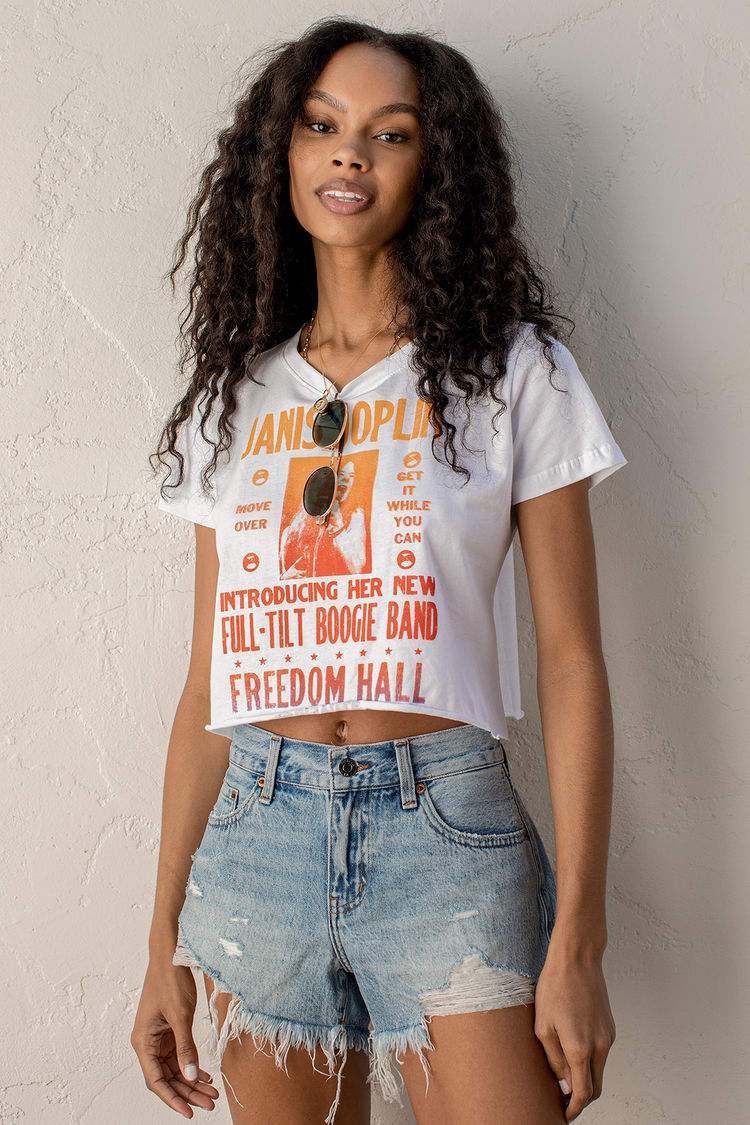The image features an African-American woman with long, curly black hair cascading down in coils, standing in front of a gray wall. She is positioned centrally and is smiling at the camera with arched eyebrows. The woman is wearing short, blue denim cut-off shorts with white trim and a white polo t-shirt. The t-shirt has bold text in orange or red that reads: "Janis Joplin Introducing Her New Full-Tilt Boogie Band at Freedom Hall." Additionally, there is a picture of Janis Joplin on the t-shirt. She accessorizes with a necklace and has a pair of black sunglasses hung on her t-shirt. The woman stands tall with her long legs and arms relaxed by her sides, exuding confidence and joy.